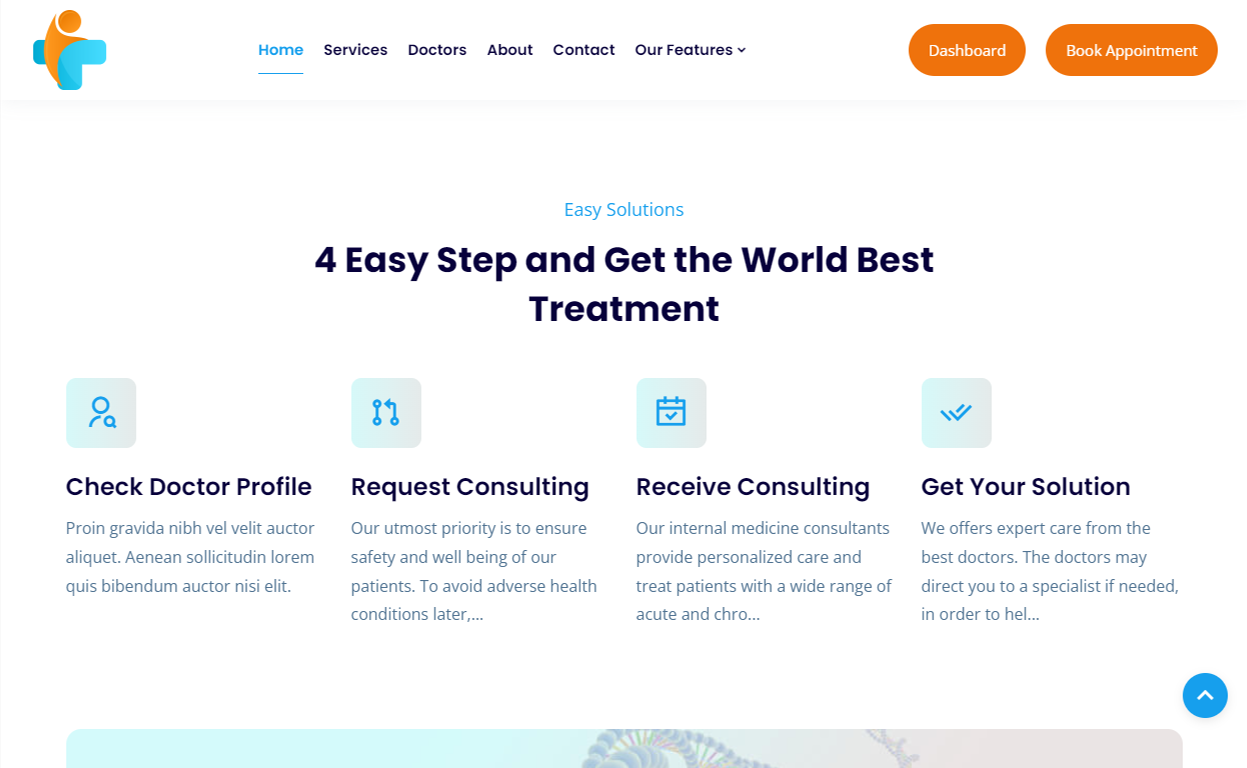This is a screenshot of a website with a minimalist design featuring a white background.

### Logo and Navigation:
Located in the top left corner is the website's logo, which depicts an abstract figure resembling a person superimposed on a blue "plus" sign. The figure's head and body are represented with an orange shape. The top menu includes six links: Home, Services, Doctors, About, Contact, and Our Features.

### Action Buttons:
Below the navigation menu, there are two prominent orange oval buttons with white text: one for accessing the Dashboard and another for booking an appointment.

### Headline and Subheadings:
The website showcases three main headlines: "Easy Solutions," "Four Easy Steps," and "Get the World's Best Treatment."

### Content Sections:
Beneath these headlines, the content is organized into columns with small icons, header texts, and detailed information. The outlined steps include:
1. Check Doctor Profile
2. Request Consulting
3. Receive Consulting
4. Get Your Solution

The text and buttons are predominantly in black and blue, with blue and orange serving as the primary accent colors throughout the design.

### Footer:
At the very bottom, there is an image partially visible that appears to be the top of a Ferris wheel, adding a subtle visual element to the footer area.